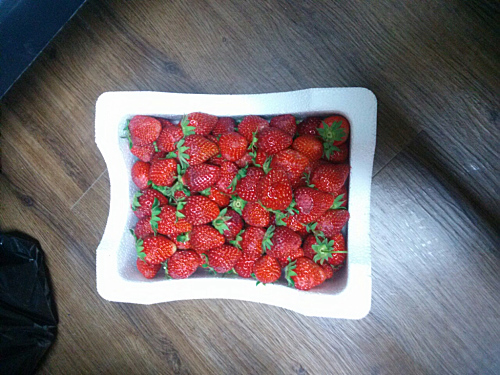This is a close-up, top-down color photograph taken indoors, showcasing a white container filled with vibrant, bright red strawberries that are piled randomly within. The strawberries, dotted with small black seeds and crowned with light green leafy tops, almost reach the top edge of the quart-sized, possibly styrofoam container. The container is rectangular with a distinctive wide curved notch on the left-hand side and another curve at the bottom, though the sides of the container are not visible due to the camera angle. The container sits on a dark brown, wood-grained floor that features distinct streaks of black. In the lower left corner of the image, an article of black clothing is partially visible, and towards the upper left corner sits a dark blue, unidentifiable object that appears to be the edge of a piece of furniture. The wood floor subtly reflects the ambient light, adding depth to the image.